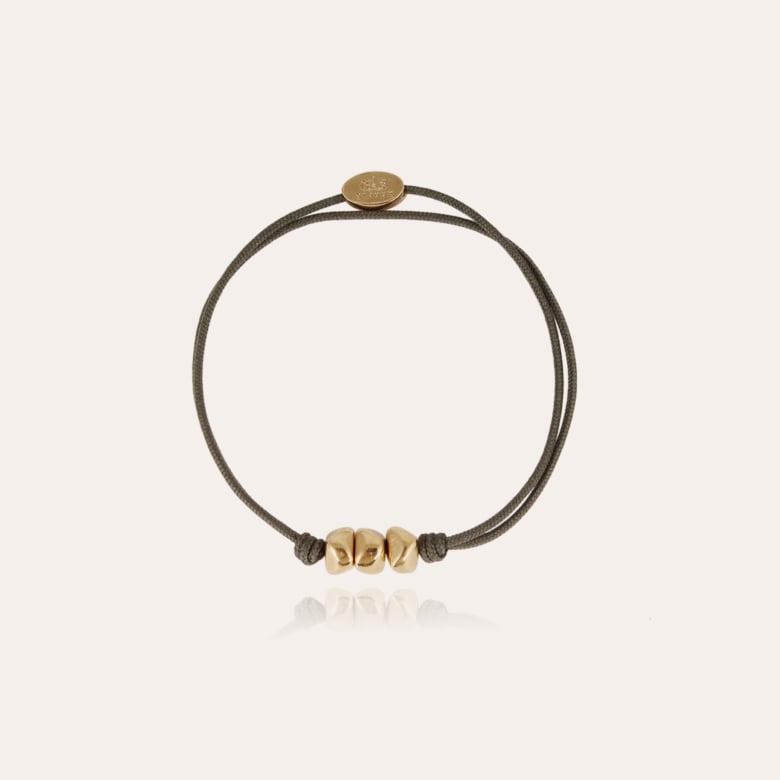The image showcases a simple piece of jewelry that could function as either a bracelet or a necklace, depending on its size, displayed against a plain white or off-white background. The jewelry is composed of two loops of gray cloth-covered elastic string or rope, which stretches slightly. The lower portion of the item features three small, golden, misshaped pebbles secured in place by knots on either side, adding a rustic, handmade charm. At the opposite end, there is a small medallion or coin, detailed with an indiscernible design due to its size. The surface below the jewelry is reflective, enabling a faint mirrored image of the piece, which gradually fades. This earthy, understated accessory exudes a sense of simplicity and natural elegance, fitting seamlessly into a higher-consciousness or minimalist aesthetic.